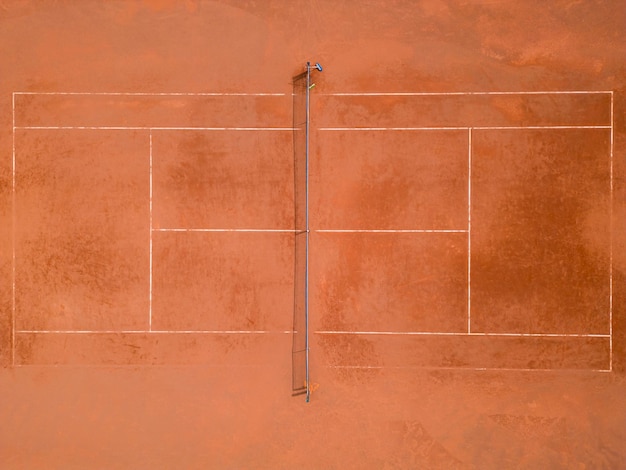This image presents an aerial view of an outdoor tennis court characterized by its distinct orange or reddish-brown surface, which has the appearance of dusty clay or red concrete. The court features standard white lines forming multiple rectangular boxes indicative of a tennis layout, although the lines appear smudged in various places, partially obscured by the dusty surface. At the center of the court, a slightly angled net stretches across, with visible shadows suggesting that the light source is coming from the right side. On the top of the net, there's a hammer-like structure that stands out. The surface of the court appears uncleansed and heavily trafficked, with traces of footsteps visible, further enhancing the impression of its dusty and worn state.